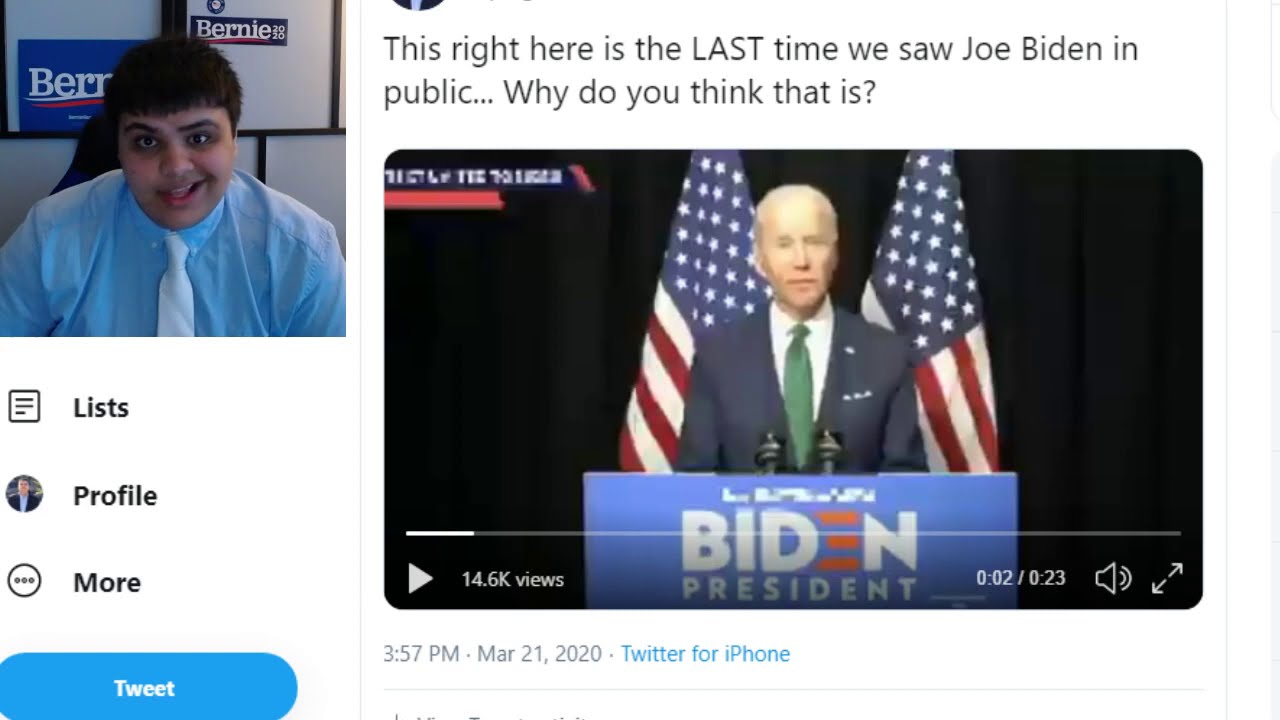The image captures a screenshot from a YouTube reaction video featuring a young man with short, dark hair, wearing a light blue button-up shirt and a white tie, seated in front of Bernie Sanders campaign stickers. His facial expression shows one eyebrow raised and his mouth slightly open. The left side of the screenshot includes his profile details, which read "List Profile More Tweet." To the right, there's a Twitter video of Joe Biden at a blue podium with his "Biden for President" logo, flanked by two American flags. The Twitter video, paused at 2 seconds of a 23-second clip, has 14.6 thousand views and is timestamped 3.57 p.m., March 21st, 2020, noted as "Twitter for iPhone." A caption above Biden's video reads, "This right here is the last time we saw Joe Biden in public. Why do you think that is?" suggesting the young man is discussing a conspiracy theory.